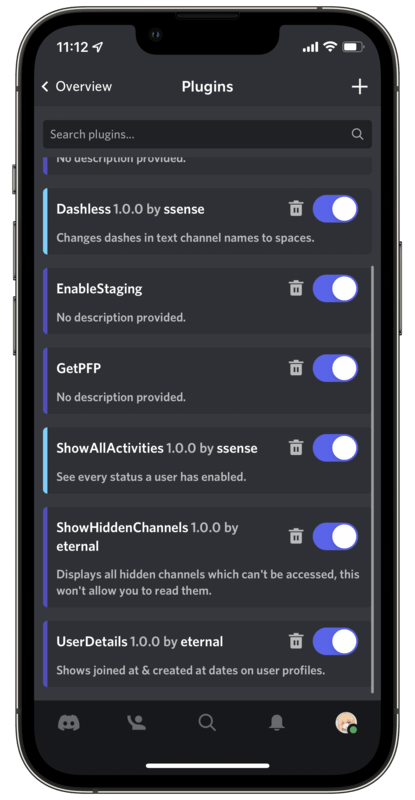The image depicts a cell phone with a prominent black screen. On the screen, the time is displayed as "11:12" in white text, situated on the top left. On the top right, there are icons showing the phone's signal bars, Wi-Fi strength, and a nearly fully charged battery.

Below the top status bar, several elements are visible:
- At the top left, a left arrow symbol is present.
- In the center, the word "Plugins" is displayed.
- On the top right, there is a plus sign "+."

Further down, a search bar is located with the placeholder text reading "Search plugins" accompanied by a magnifying glass icon, indicating a search function.

Below the search bar, there is partially visible script that reads "no description provided," which appears to be cut off.

Continuing downwards, the following details can be seen:
- "dashes-dashless 1.0.0 by CENSUS" with an "SE" label next to it. This item features a blue toggle indicating it is enabled, alongside a trash can icon. The functionality described is to "change dashes in text channel names to spaces."
- Another section reads "enable staging," again marked with "no description provided" and a blue toggle indicating it is on. A trash can icon is present here as well.
- "Get PFP" appears with no additional description, a trash can, and a blue toggle indicating it is activated.
- "Show all activities 1.0.0 by CENSUS," which is described as allowing the user to see every status a user has enabled. This section also shows a trash can and a blue toggle indicating it is active.
- The bottommost visible section starts to describe "Show hidden channels 1.0..." but is cut off.

Each of these sections includes a blue toggle switch and a trash can icon, suggesting options that can be enabled/disabled or deleted.